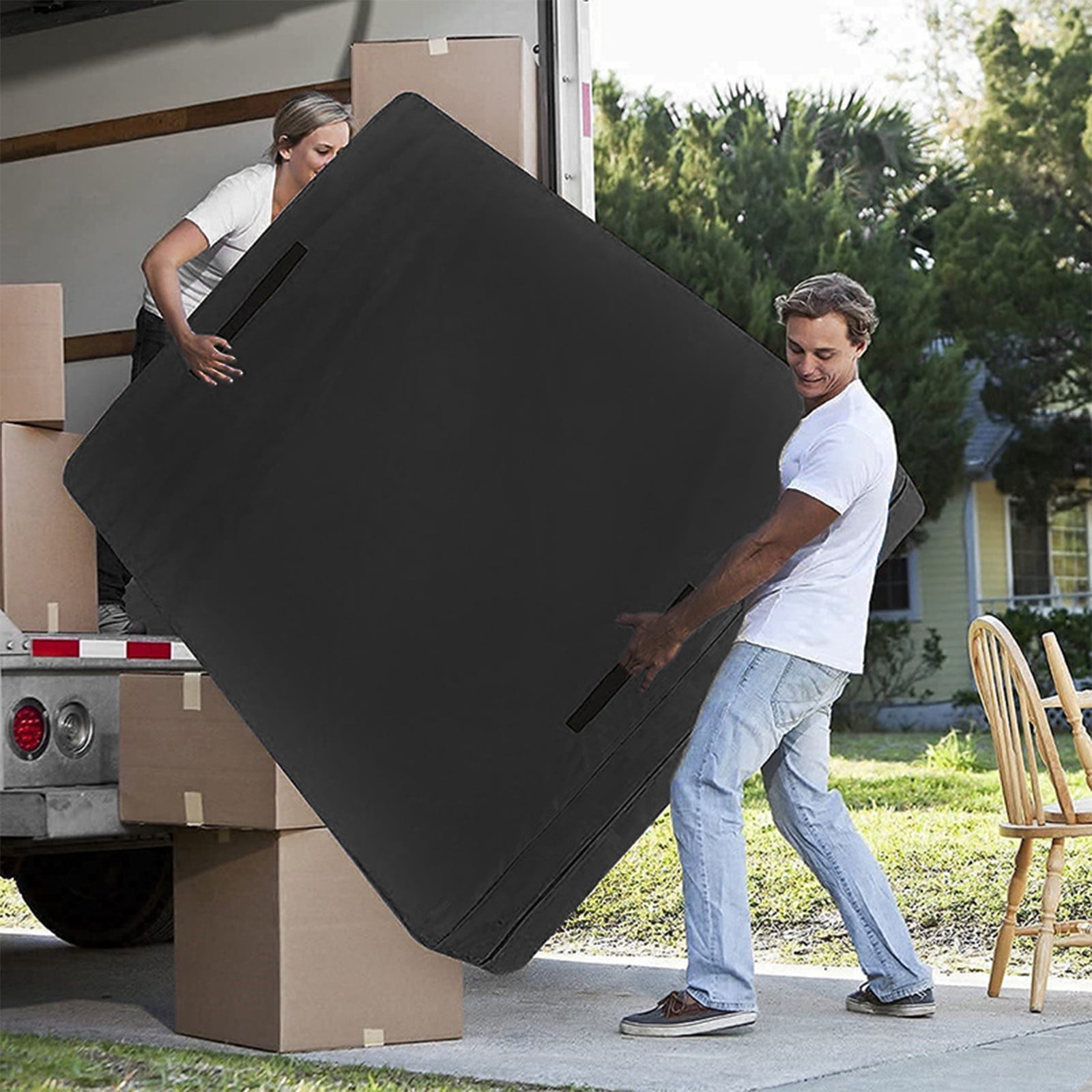In this image, two individuals are engaged in loading a moving truck. The scene features a well-built Caucasian man, identifiable by his short hair, wearing a white t-shirt, light gray-blue jeans, and brown boat shoes. He is on the right side of the image, seemingly holding the bottom portion of a large, black rectangular cushion, which resembles a mattress. 

Inside the moving truck, positioned on the left side of the image from the upper portion to the lower, stands a woman. She sports a white t-shirt and black pants and is assisting by holding the upper side of the same black cushion. 

The realistic nature of the image is questionable; the coloring appears unnatural and mismatched, particularly the man's hand and face tones, leading to speculation that it might be digitally manipulated. The surroundings confirm a moving scenario, with several boxes both inside and outside the truck. Tan, wooden chairs can be seen on the concrete driveway, and in the background, there's a house with yellow siding and pine trees, indicating a residential move.